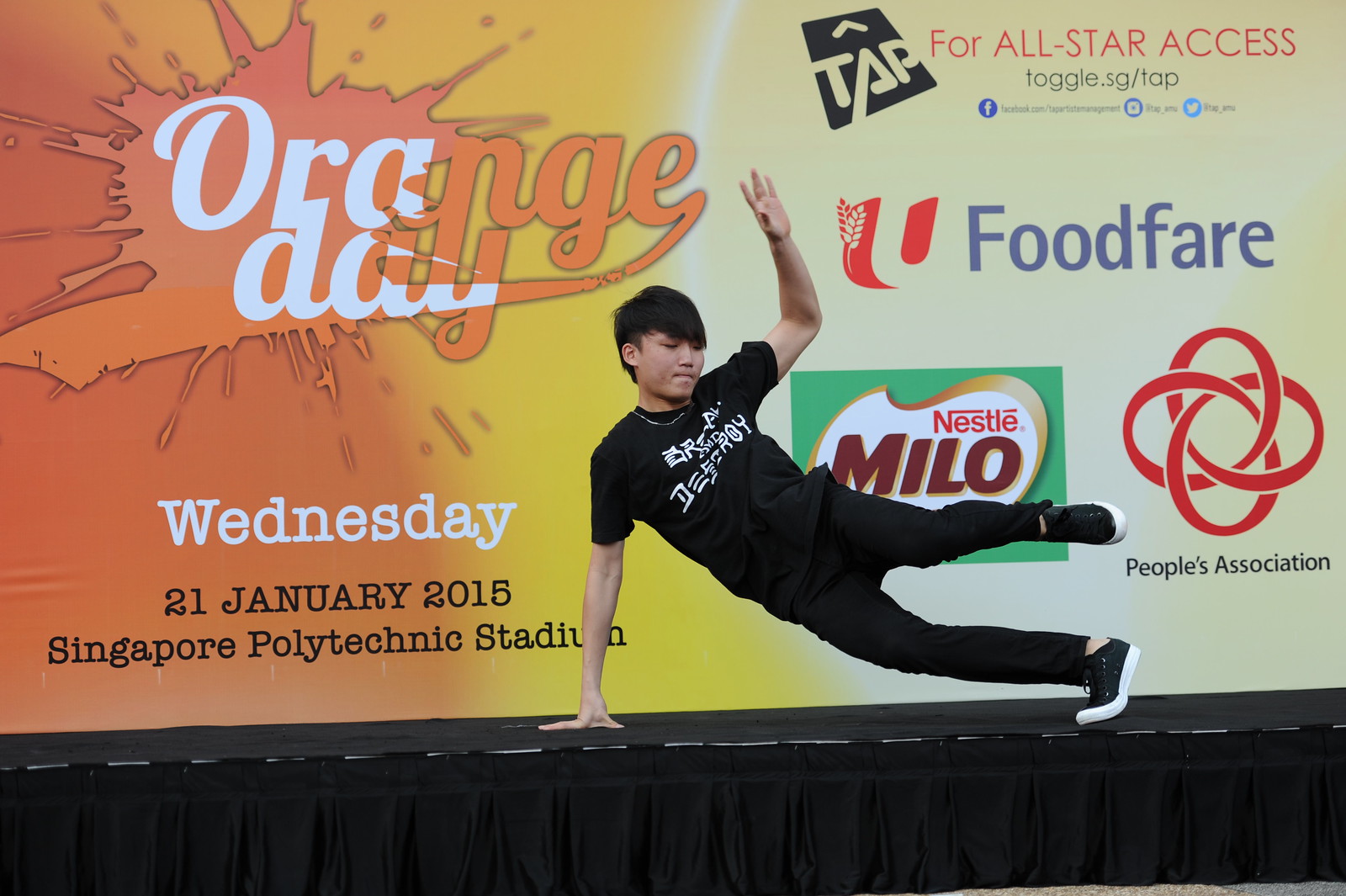This detailed photograph captures a young Asian male, approximately 14 or 15 years old, performing a captivating b-boy breakdancing move on stage. He's dressed in a black t-shirt with white text, black jeans, black sneakers with white soles, and potentially a necklace. The dancer is parallel to the ground, supported by his right arm, which is extended with his palm flat on the dark stage floor. His left arm is raised with a bent elbow, and his left leg is elevated and extended behind him while his right foot supports his weight, twisted on its toes.

The backdrop is a large billboard promoting an event named "Orange Day", featuring an orange-to-yellow gradient background on the left. The text "Orange Day" is displayed in a mix of white and orange lettering, followed by the event details: "Wednesday, 21 January 2015" in black text, and "Singapore Polytechnic Stadium." On the right side of the billboard, there is a tan background with multiple advertisements and logos. In the upper right corner, the red text reads "For All Star Access," followed by the blue text "toggle.sg/tap" and social media icons for Facebook, Instagram, and Twitter. Nearby, a tilted black square contains the initials "TAP." Additional logos include Foodfare with a tan branch design, Nestlé Milo featuring a green background with a white center and gold outline, and the People's Association logo, consisting of a red geometric symbol and black text. The overall scene captures the energy and promotional spirit of the Orange Day event.